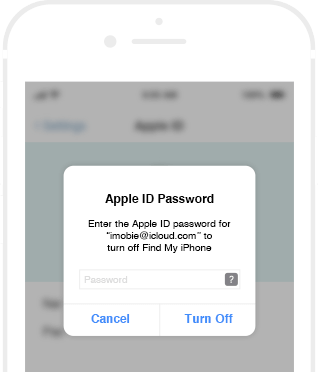A detailed and cleaned-up caption for the image could be:

"A graphic representation of a smartphone displaying a screenshot where an Apple ID password prompt appears. The graphic features a minimalist outline of a phone, and within the screen area, there's a clear screenshot. The pop-up notification reads, 'Apple ID Password,' and prompts the user to 'enter the Apple ID password for imobie.icloud.com to turn off Find My iPhone.' A text box for password input is accompanied by a small gray question mark button on the right. Below the text box are two blue buttons labeled 'Cancel' and 'Turn Off.' The pop-up slightly obscures a blurred background showing a partial view of a previous screen, revealing a white top banner, a light blue section, and another white section with blurred black text. The background includes varying shades of blue, ranging from dark blue to turquoise."